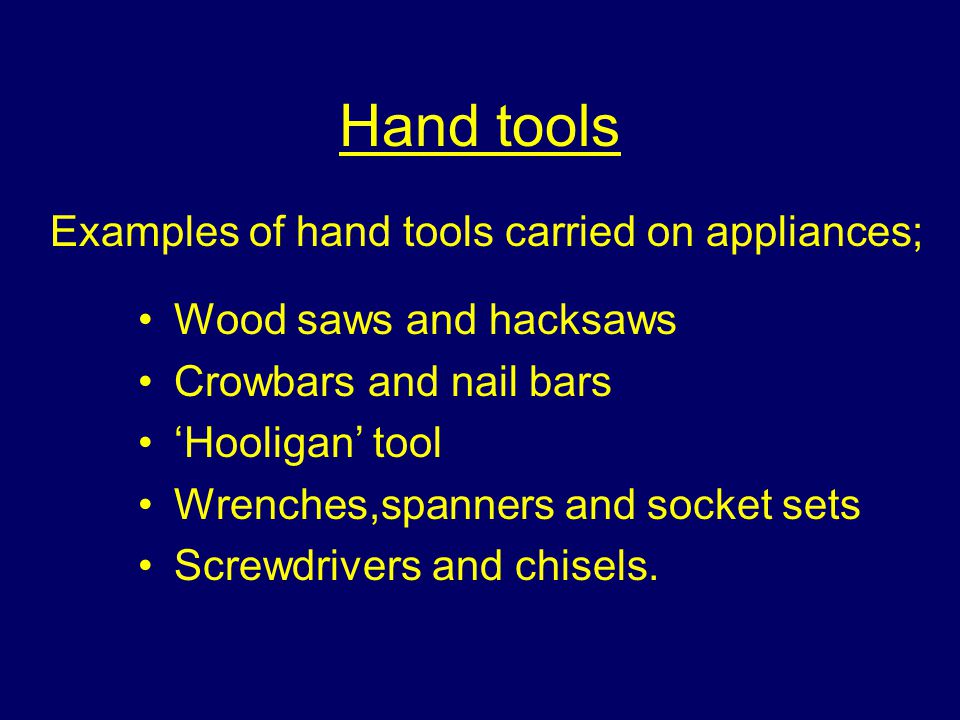The image depicts a sign with a dark blue background and yellow text. The title "Hand Tools" is prominently displayed at the top, with "Hand" in capitalized H and the rest in lowercase letters, and it is underlined. Below the title, the sign reads "Examples of hand tools carried on appliances;" followed by a list of items presented as bullet points. The list includes: 

- Wood saws and hacksaws
- Crowbars and nail bars
- Hooligan tool (with "Hooligan" in parentheses)
- Wrenches, spanners, and socket sets
- Screwdrivers and chisels

All text on the sign is centered and in yellow. The layout and presentation suggest it may be a PowerPoint slide or a computer-generated sign intended for workers, detailing the necessary hand tools to be carried on appliances.